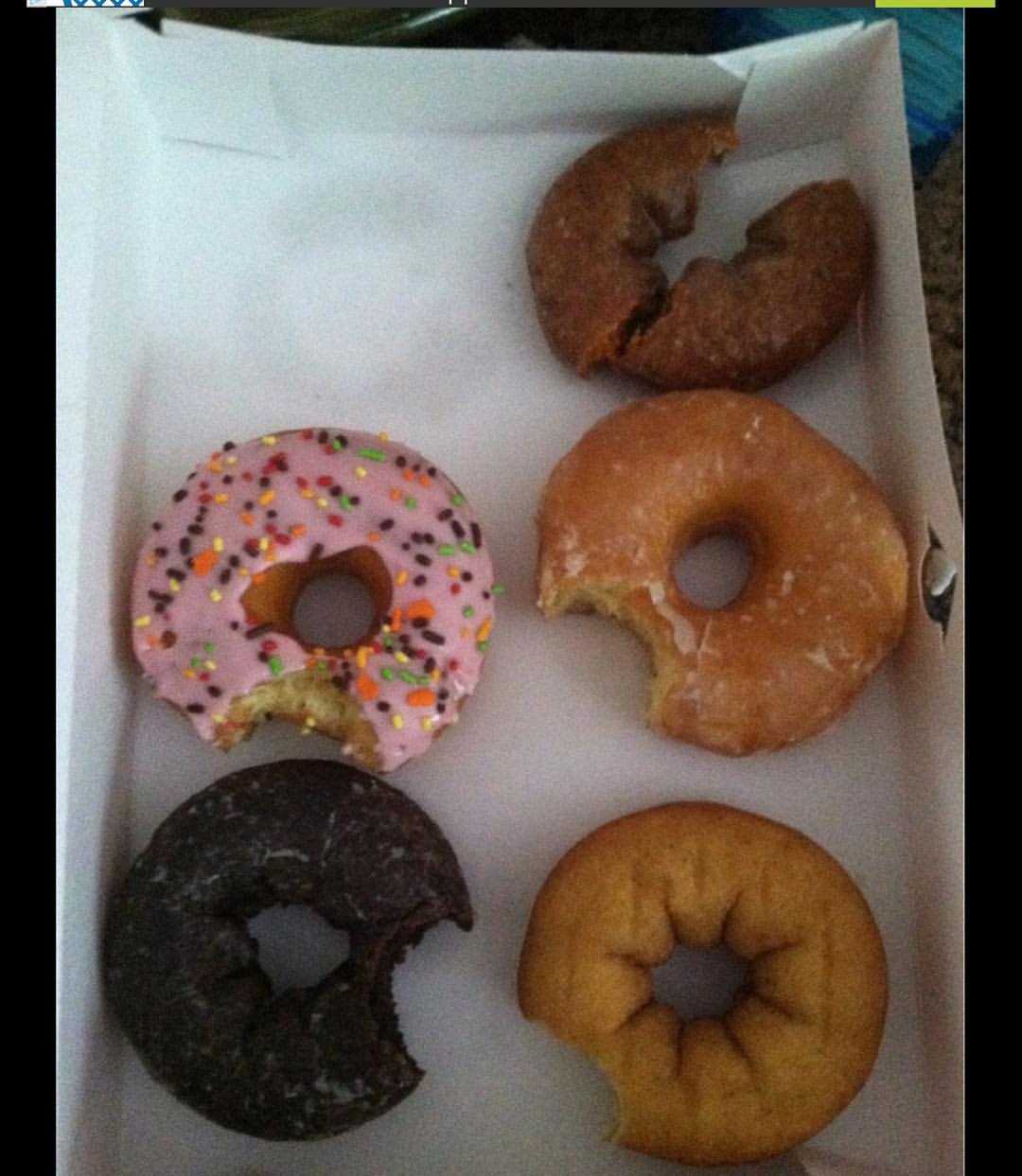The photograph shows a top-down view inside a white cardboard donut box, sitting on what appears to be a Formica counter. It contains five ring donuts, and all of them have a bite taken out of them. The poor quality of the image suggests it was taken with an older or low-resolution camera, with grainy, pixelated aspects and poor lighting. There's evidence of a missing sixth donut from a grease mark in the box. 

The assortment includes: 
1. A pink frosted donut with multicolored sprinkles (orange, yellow, green, and brown) in the middle left.
2. A dark chocolate-glazed donut in the bottom left.
3. A plain ring donut in the bottom right. 
4. A regular glazed donut in the middle right.
5. A donut in the top right that is broken in two, appearing to be a mid-brown cake type, possibly cinnamon or blueberry.

All the donuts show signs of having been partially eaten, adding a whimsical yet slightly chaotic vibe to the image.